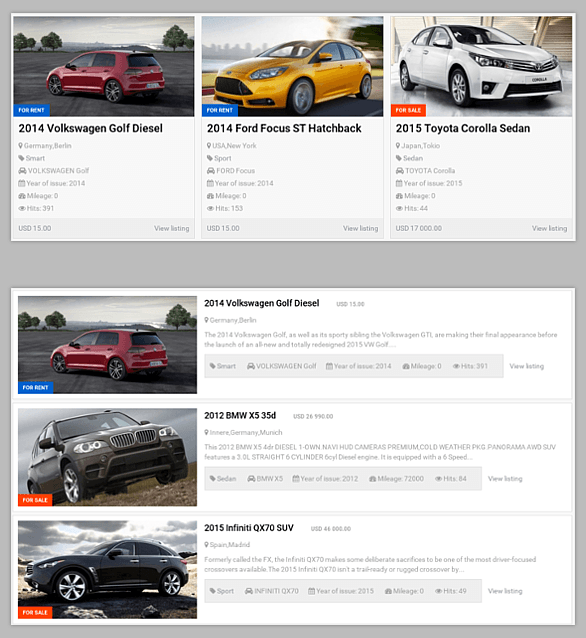The image displays what appears to be a well-lit showroom featuring miniature car models. The first row showcases a vibrant red 2014 Volkswagen Volk Diesel, followed by a sleek Ford Focus S2 Hatchback, and a pristine white 2015 Toyota Corolla Sedan. Each model's details are clearly visible and they are arranged neatly side by side. The words "For Rent" are prominently displayed in blue text next to the first two cars, while the 2015 white Toyota Corolla is marked as "For Sale."

Below, three more car models are aligned vertically. The top one is another 2014 Volkswagen Volk Diesel, followed by a refined 2012 BMW, and finally, a sophisticated 2015 BMW. The layout and labeling are clear, making it easy to distinguish between the rental and sale options.